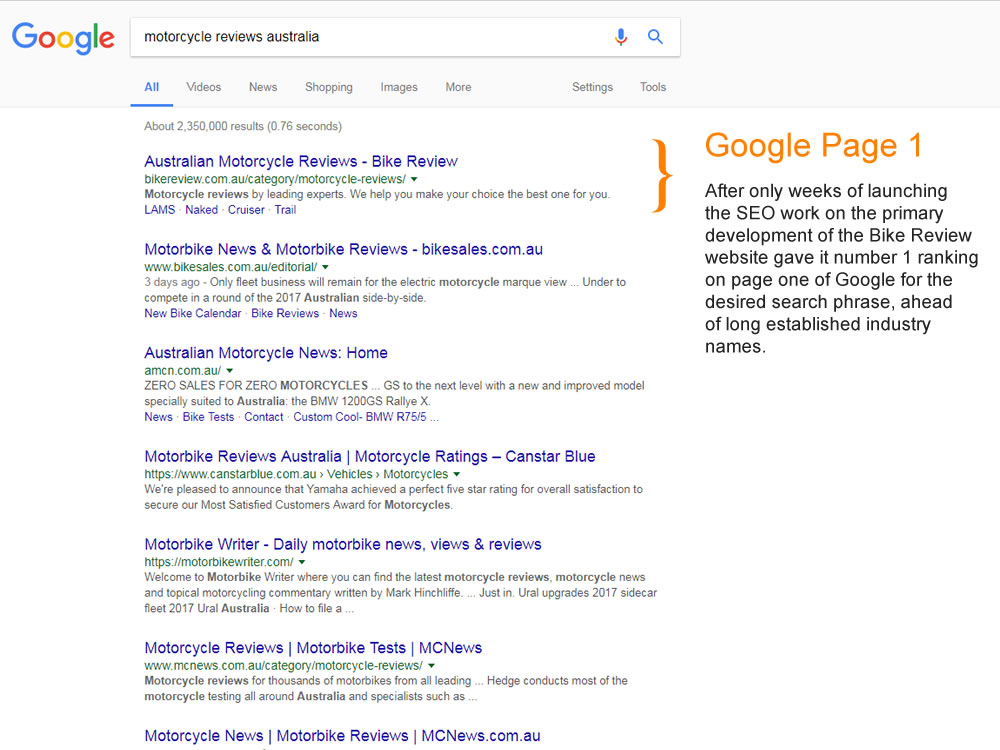Here's a cleaned-up and detailed caption for the image:

---

This image captures an older version of a Google search results page, identifiable by its traditional rectangular search bar, which predates the more contemporary oval design. The search query "Motorcycle Reviews Australia" is prominently displayed at the top in black text. Beneath the search bar, several navigational tabs are visible, including "All," "Videos," "News," "Shopping," "Images," and "More," with "Settings" and "Tools" positioned on the far right.

The page indicates approximately 2,350,000 results found in a swift 0.76 seconds, as noted in small grey text. The first search result is titled "Australian Motorcycle Reviews—Bike Review," highlighted in blue. This particular result is accented with an orange bracket to the right. Above this bracket, in a rounded sans-serif font and orange text, it reads "Google Page 1." 

Below the title, in smaller black text, it states: "After only weeks of launching, the SEO work on the primary development of the Bike Review website gave it number one ranking on page one of Google for the desired search phrase, ahead of long-established industry names."

Subsequent listings follow, each in blue text:
1. "Motorbike News & Motorbike Review—Bikesales.com.au"
2. "Australian Motorcycle News: Home"
3. "Motorbike Reviews Australia"
4. A line separates the following listing: "Motorcycle Ratings—CanStarBlue."

---